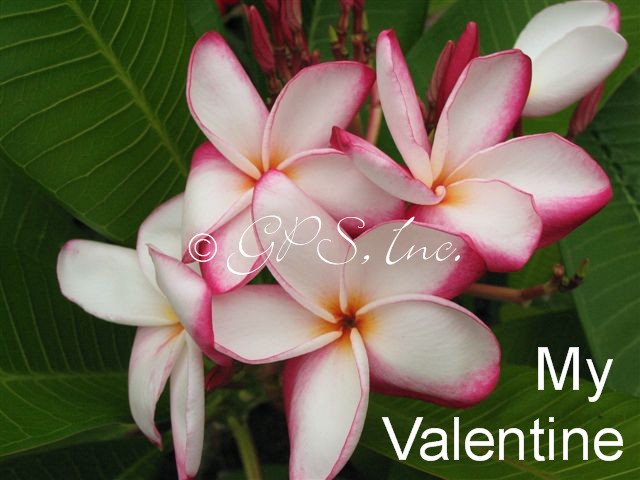The image showcases a stunning close-up of a bunch of five delicate white and pink flowers that resemble orchids, often found in Hawaii for their strong scents. Each flower, with five petals, features bright pink edges contrasting against vibrant green leaves. Behind the flowers, additional buds hint at more blooms to come. The scene is set against a blurred background, emphasizing the flowers' beauty. At the center of the image is a watermark that reads "© GPS Inc.," while the bottom right corner features the white text "My Valentine," with "My" positioned above "Valentine," suggesting this picture might be part of a Valentine's Day card, highlighting the meticulous and high-quality presentation.